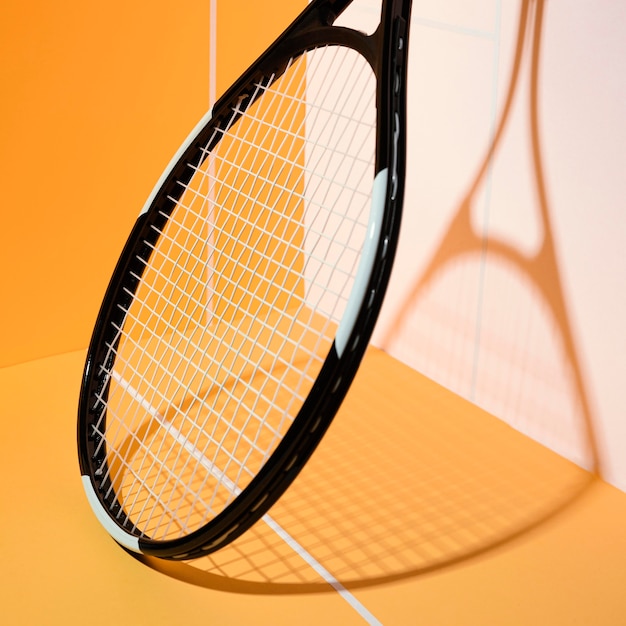This detailed image captures a close-up of a black tennis racket with white strings, set in an orange and white room that evokes the setting of a tennis or racquetball court. The scene is set in a corner where the right wall is white, and the left wall and floor are a peachy orange color, both featuring white stripes. The racket rests at an angle with its handle propped against the orange wall and the stringed section touching the floor, creating an intriguing shadow on the white wall that vaguely resembles the Eiffel Tower. The lighting comes from the left, enhancing the shadow and adding depth to the image. The image is devoid of any text, allowing the vibrant colors and composition to take center stage.